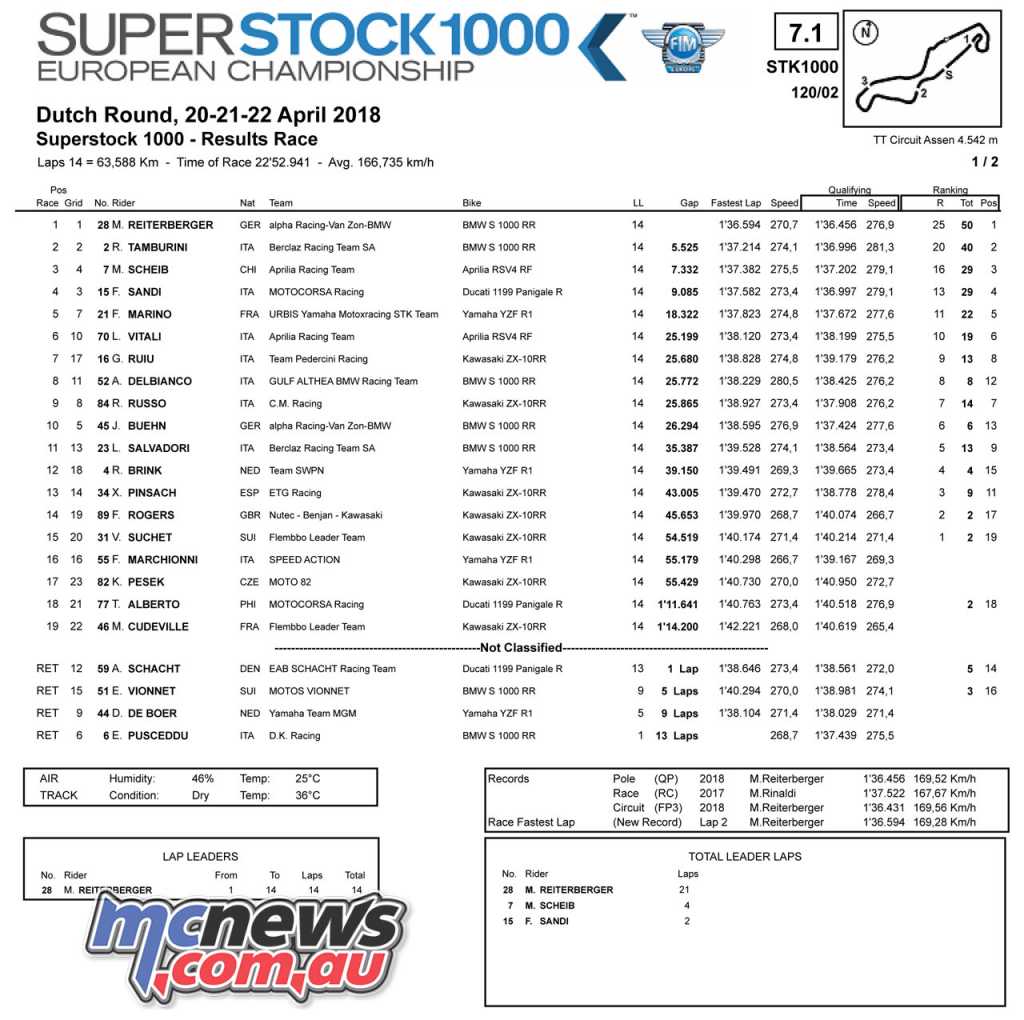This image, resembling an informational handout or pamphlet, showcases the detailed results of the Super Stock 1000 European Championship Dutch Round held on April 22, 2018. In the top left corner, "Super" is printed in gray, and "Stock 1000" follows in blue, with "European Championship" stated just below. Directly to the right appears a rudimentary track outline and beneath it a box labeled "Wings." The event title is reiterated as "Super Stock 1000 Results Race," highlighting details such as 14 laps, race distance in kilometers, time of race, and average speed.

Structured in a well-centered table format, the handout lists the racers from positions 1 through 19, documenting their grid placement, rider names, nationalities, teams, bike types, lap speeds, and gaps among other metrics. There's an additional section labeled "Not Classified," starting with the abbreviation "RET," listing riders and corresponding data not included in the main results. 

Towards the bottom, additional data is provided in two boxes on the right, displaying figures relevant to the race, and a box on the left specifying air temperature, track condition, and humidity levels. The color scheme of the document includes shades of gray, blue, black, white, and accents of red. Finally, the bottom left corner features the logo "mcnews.com.au," with "MC" in blue, "News" in black, and the remainder in red.